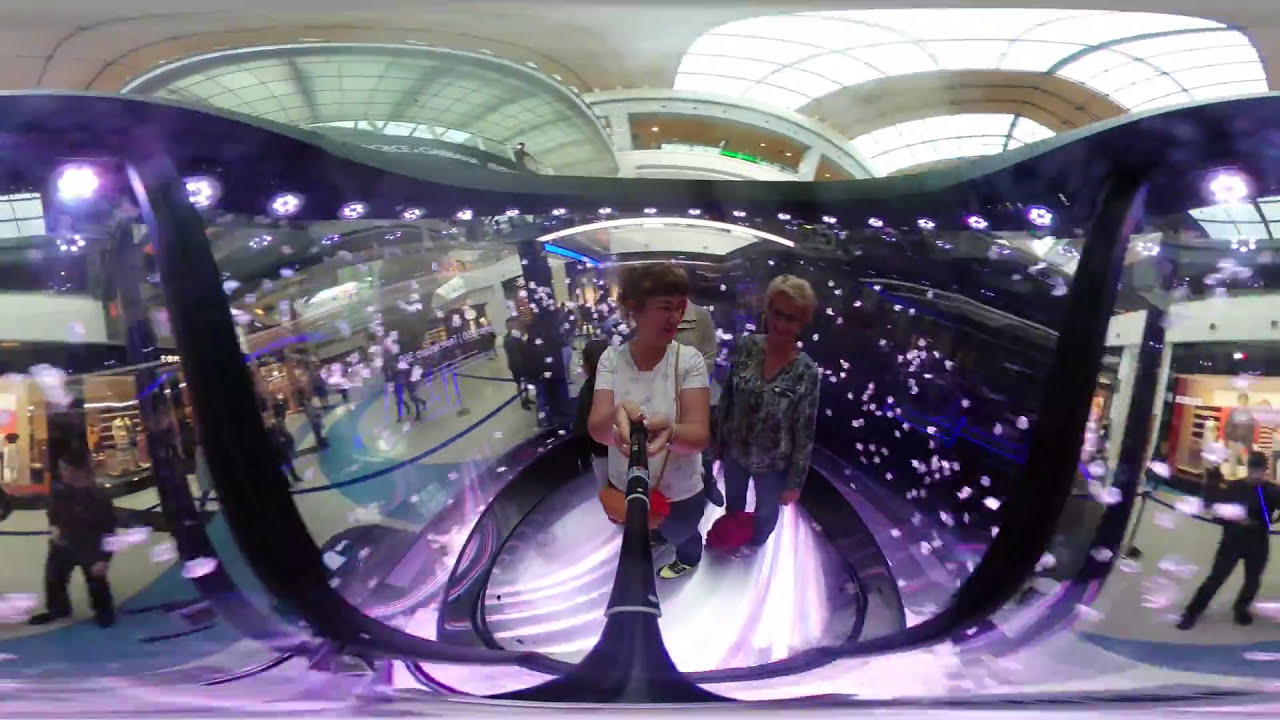The image captures a bustling indoor scene, likely within a mall, with white and blue-tiled flooring and a white ceiling with windows allowing natural light to stream in. Amidst the crowd, two women stand prominently in the center. The woman on the left is middle-aged, with brown hair, wearing a white t-shirt with a design, blue jeans, white and black shoes, and a brown crossbody purse. She holds a black selfie stick with a device that has white lights facing inward. The blonde woman next to her is dressed in a green and white collarless shirt with blue jeans. She has a red, possibly maroon, bag positioned between her legs. The background reveals department stores on both sides, with people in dark clothing walking about, and a line of mannequins visible in the store windows. A blue rope with pegs is seen, indicating a queuing area. Both women appear to be sharing a moment, possibly taking a selfie together, amidst the vibrant mall environment.